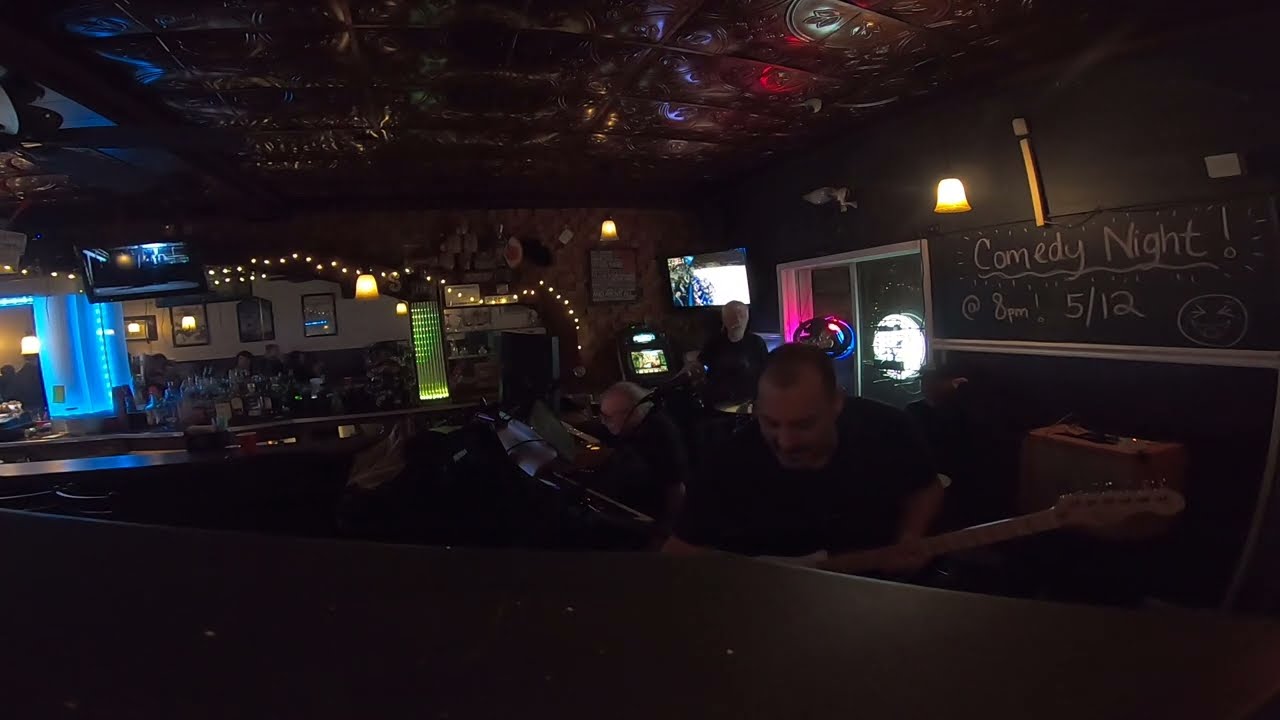The image depicts the dimly lit interior of a club or bar with a cozy, tavern-like atmosphere. On the right wall, there's a partially illuminated chalkboard banner that reads "Comedy Night! 8 p.m. 5/12" in large, silver freehand letters with a squiggly underline and a smiley face. Above the banner, a yellow wire leads to a lightbulb, casting a warm glow. To its left, another lightbulb emits more yellow light, creating a heavy circle of illumination at the bottom. Below the banner, a brown leather couch accommodates several people, including a Caucasian man with a receding hairline holding a guitar part and reaching over the couch’s back.

On the left side, fluorescent blue lights illuminate the white back wall, where four framed pictures hang, reflecting both blue and yellow light. A square TV screen hangs straight on the back wall, showing an image with a white bottom and dark top. In front of the TV stands a man in a black shirt with gray hair. A string of yellow lights stretches from the left across the room, ending near a green and yellow cylinder-shaped light.

Patrons are scattered throughout, sitting at tables and benches, many with drinks. In the foreground, nearly invisible due to the dimness, others sit at a curved bar. Decorative Christmas lights and tulip-shaped lamps add to the festive ambiance. The overall scene is quite dark, making it difficult to see many details clearly, but the cozy and intimate atmosphere of the club is palpable.